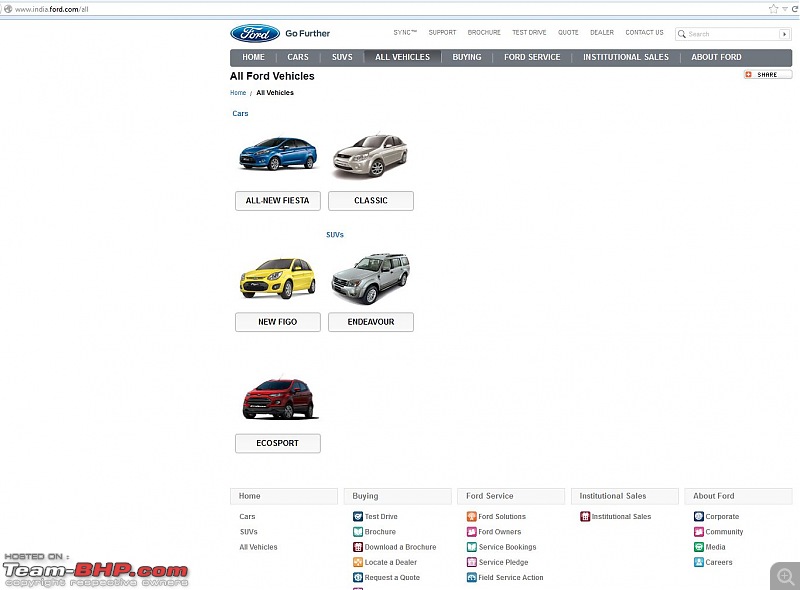This screenshot captures the homepage of Ford’s website, showcasing a diverse range of Ford vehicles including the all-new Fiesta, Figo, Endeavour, and EcoSport. Upper sections of the page feature several menu options such as 'Home,' 'Cars,' 'SUVs,' 'All Vehicles,' 'Buying,' 'Ford Service,' 'Institutional Sales,' and 'About Ford.' Beneath these categories are various icons and clickable links for easy navigation. The top left corner displays the Ford logo, while the top right corner includes a search bar for quick access. Additionally, the website URL, Ford.com, and the external link TeamVHP.com are clearly visible.